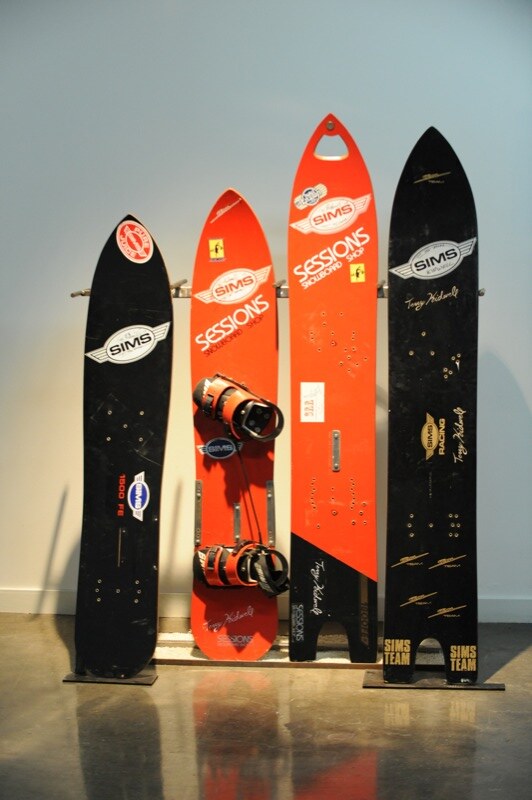This color photograph captures four vertically positioned snowboards, two bright orange ones in the center flanked by black ones on both sides, all set against a bluish wall. Each snowboard prominently features a white Sims logo. The two middle orange snowboards also display an additional Sessions logo beneath the Sims branding, accompanied by the words "Snowboard Shop" and a small yellow symbol. Unique among them, the leftmost snowboard is equipped with attached boots, unlike the others, which have visible holes for boot attachment. The reflective polished stone floor below mirrors the snowboards, enhancing the sleek, organized presentation. The black snowboards have additional less legible logos and signatures towards the bottom, with one featuring an orange and bluish logo and the other a yellowish one. Overall, the image encapsulates a well-arranged display of snowboarding gear in a polished environment.